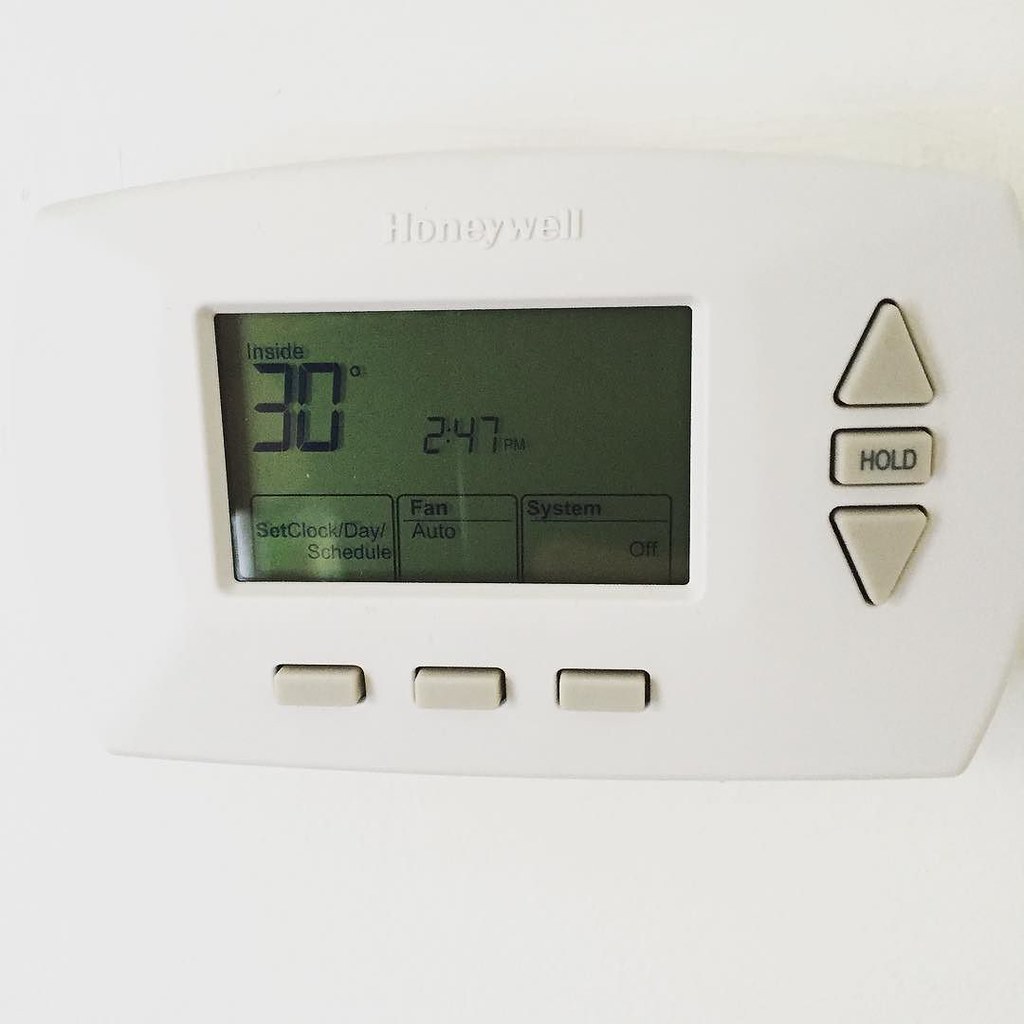The image features a sleek, all-white Honeywell thermostat prominently engraved with the brand name "Honeywell." At the center of the device is a square digital screen displaying various details. The screen shows the word "Inside" followed by the current temperature, marked as "30°," with the degree symbol situated at the upper right corner of the zero. The time displayed is 2:47 p.m. 

Beneath the temperature and time readout, there are three small squares within the digital interface. The first square reads "Set Clock/Day/Schedule," the second labeled "Fan" and "Auto," and the third reads "System" with the word "Off" beneath it. Below the screen, three tiny gray buttons line up horizontally. On the right-hand side of the thermostat, there is a vertically aligned set of buttons, including a triangle-shaped button, a rectangular button marked "Hold," and an inverted triangle button. The entire device is mounted against a clean, white wall.